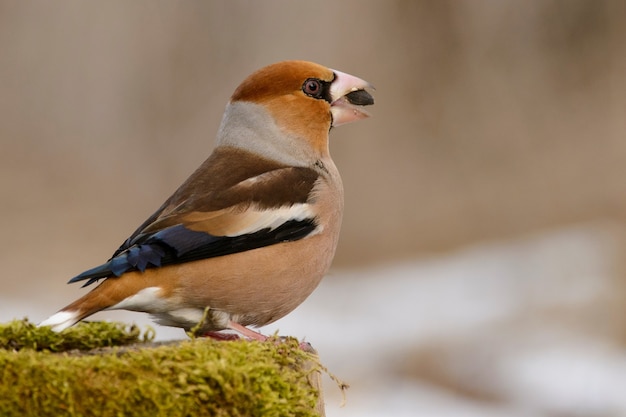The photograph captures a small bird perched on a green mossy rock, its profile facing to the right. The bird features a striking orange head, with a white neck transitioning into a white back, and brown feathers further down. Its wings are a mosaic of white on top and black, with a touch of tan. The underbelly is tan, and the tail is brown with a white tip, complemented by white underneath. Its feet are notable with pinkish skin. The bird's beak is tan with what appears to be a large black object, possibly food, sticking out. Its eyes are a vivid orange with black centers, giving it a healthy and plump appearance. The backdrop is a mix of tan and brown blurs, indicating a shallow depth of field which keeps the focus securely on the bird.